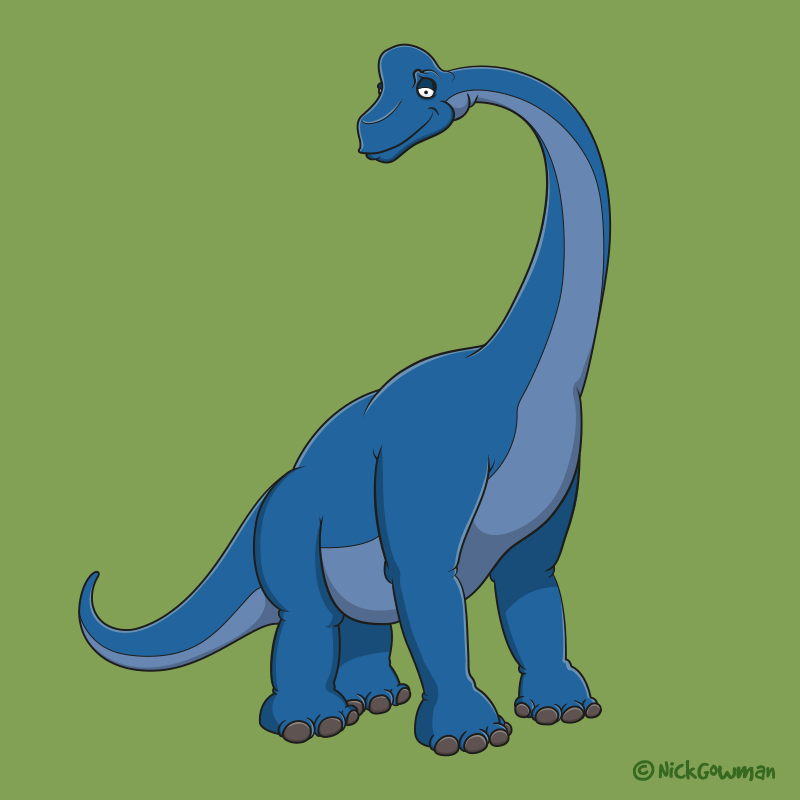The image is a vibrant cartoon drawing of a long-necked dinosaur, possibly a Brontosaurus or a similar species. The dinosaur is predominantly dark blue with a light blue underbelly, extending from its neck down to its tail. It features a squared snout, a small crest atop its head, and has four visible toes on its front feet and three on its back feet. The creature's lazy eyes, adorned with white sclera and small dot-like pupils, look upwards and slightly to the left. The background is a forest-like green, blending olive and pea green shades. In the lower right corner, there's a green copyright symbol followed by the text "Nick Gohmann," indicating the artist responsible for this colorful depiction.